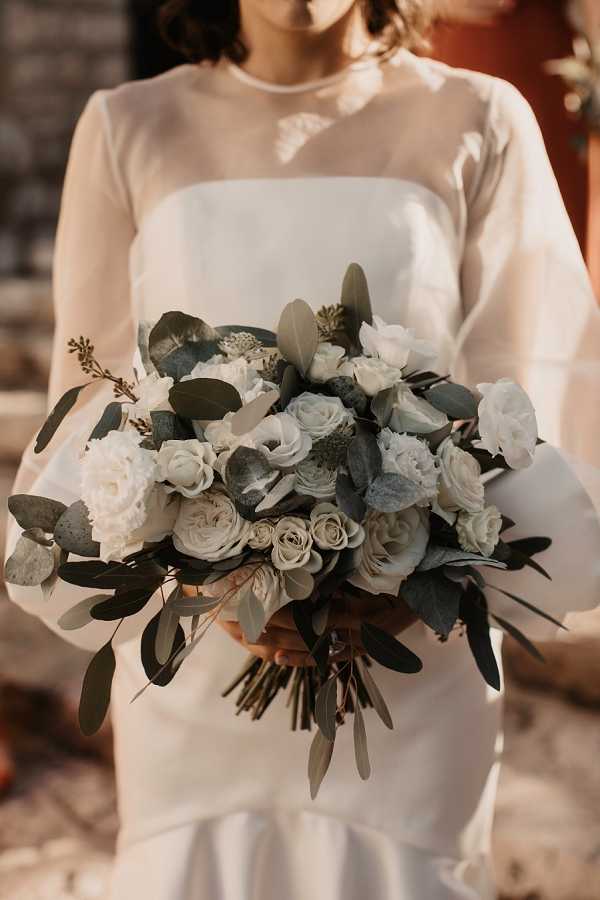In the image, a white-skinned woman with shoulder-length dark brown hair is seen from just above her knees to beneath her chin. She is holding a large bouquet of flowers in front of her, obscuring her hands. The bouquet consists of white and gray roses interspersed with dark olive green leaves, and hints of fern-like foliage. The woman is dressed in a white gown. The dress has a see-through fabric from above her chest, revealing her shoulders and arms, making it appear as if she is wearing a strapless dress with sheer long sleeves. Below the chest, the dress is opaque, extending down to her knees with a visible sewn hemline and subtle wrinkles. The out-of-focus background on the right side shows a light pink hue, while the left side has a dark spot that is indistinguishable, next to what appears to be part of a gray stone or brick wall. The overall composition draws attention to the bouquet she is holding, suggesting a bridal or bridesmaid context.